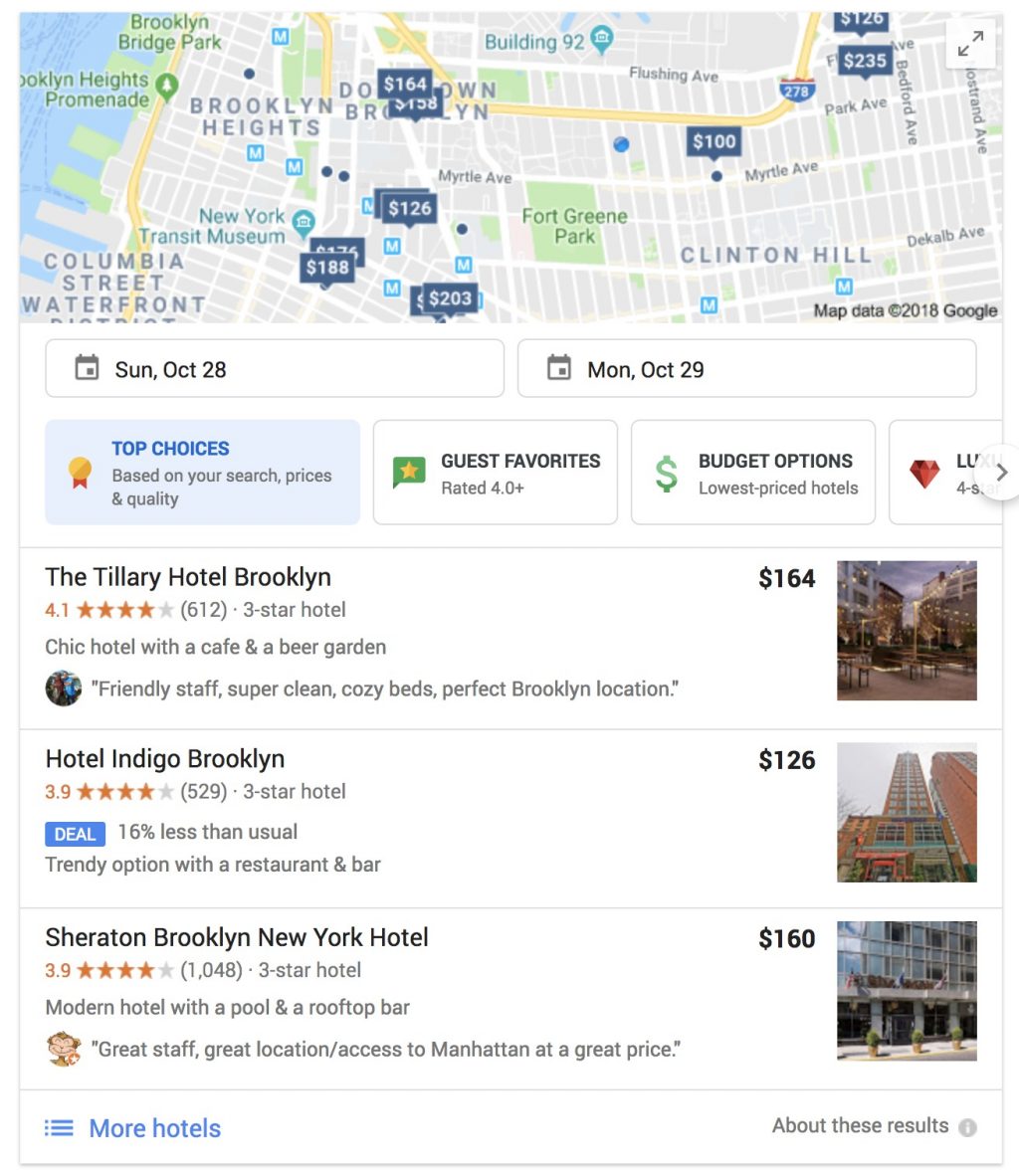This detailed caption provides a comprehensive description of a visual image of a map, focusing on various geographic and commercial highlights within Brooklyn, New York:

"The image illustrates a detailed map of Brooklyn, New York, highlighting significant locations including Brooklyn Heights, the New York Transit Museum, Brooklyn Bridge Park, and the Brooklyn Heights Promenade. Key areas like Columbia Street Waterfront and Clinton Hill are also marked. The map features numerous blue squares displaying various figures in white, such as 4, 126, 182, 103, 100, 235, and 126, which appear to denote prices or data points.

The map also shows metro routes marked with gray squares and a prominent yellow highway. Building 92 on Flushing Avenue and Myrtle Avenue are identified. In the center of the map is a park, with additional notations indicating dates, saying 'Sunday, October 28th, Monday, October 29th.' This visual seems to tailor choices based on search criteria, quality, and pricing, highlighting 'Top choices,' 'Guest favorites rated 4.0+,' 'Budget options,' and 'Lowest priced hotels.'

Prominent hotel recommendations include:
- The Tillery Hotel Brooklyn, rated 4.1 stars (612 reviews), described as a chic, three-star hotel with a cafe and beer garden, praised for its friendly staff, cleanliness, and cozy atmosphere.
- Hotel Indyville Brooklyn, noted as a trendy option with a restaurant and bar, priced at $26.
- Sheraton Brooklyn New York Hotel, a modern hotel featuring a pool.